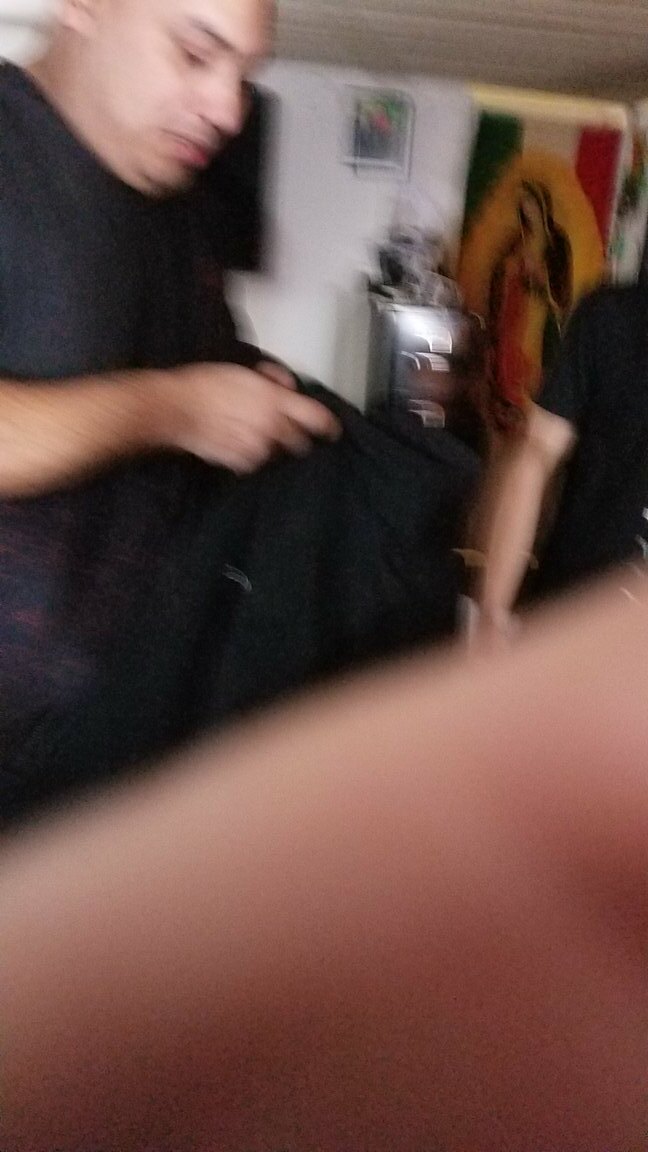In this blurry indoor photograph, captured in a residential setting, two light-skinned individuals dressed in black attire are depicted. The image is mostly vertical, with a finger obscuring the lower portion. On the left, a bald man faces right, partially visible and wearing a black t-shirt and dark pants. He holds an indistinct dark object at chest level, potentially blending into his attire. To his right, another individual, cropped and less visible, reveals only a right arm and part of a black t-shirt. The background features white walls adorned with a flag turned sideways, displaying green, white, and red horizontal stripes. Prominently, an oval picture of the Virgin Mary overlays the flag. Nearby, another indistinct picture is present on the wall.